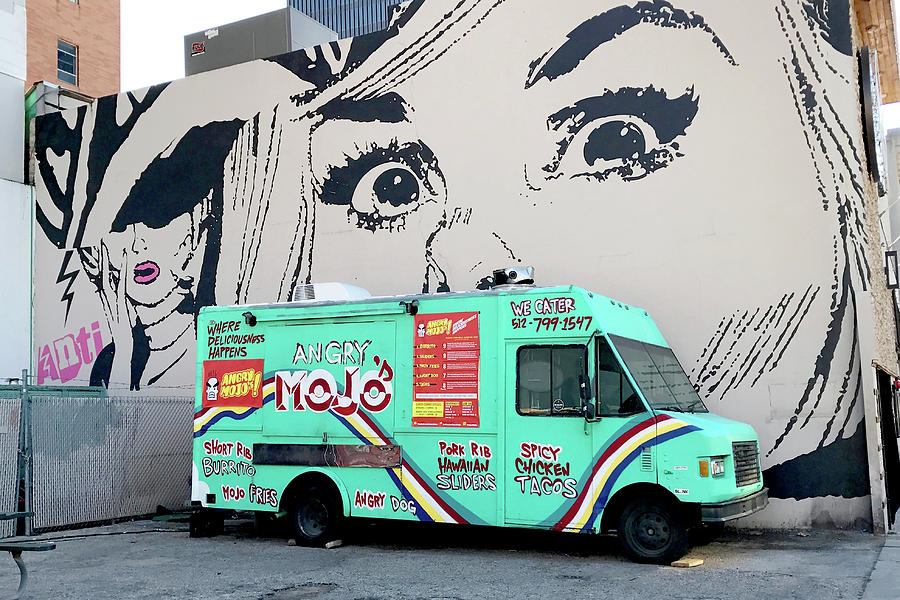The image features a lime green vending truck labeled "Angry Mojos" with the tagline "Where Deliciousness Happens." The truck advertises a menu including Spicy Chicken Tacos, Pork Rib Hawaiian Sliders, Short Rib Burrito, Mojo Fries, and Angry Dog, and offers catering services with a contact number 512-799-1547. The truck is parked in front of an urban building adorned with striking murals. One mural showcases a woman with large, expressive eyes and a startled expression, rendered mostly in black and white with pink highlights. To her left, another figure of a woman is depicted wearing a darkly shadowed, ornate hat, her hand resting on her cheek. This second mural features vivid pink lips and the word "ANTI" signed in pink text. The artistic style resembles 1950s pop art, evoking elements of Andy Warhol’s work.